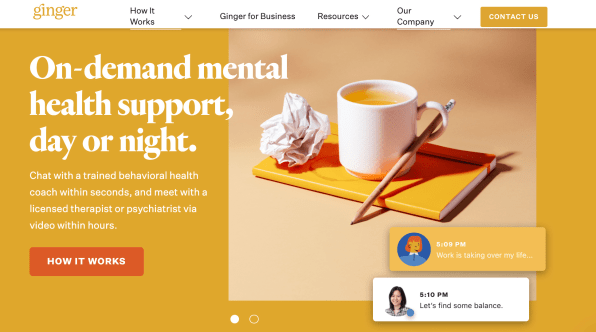This visual representation of the Ginger webpage showcases an interface designed with a gold-toned theme. Dominating the page is a large gold square, seamlessly integrating various elements. At the peak of the page, the brand name "Ginger" is prominently displayed in gold lettering. Nestled in the top left corner, black text guides visitors through different sections: "How It Works", "Ginger for Business", "Resources", "Our Company", and "Contact Us."

The core feature of the page is a powerful slogan centered in bold white text: "On-Demand Mental Health Support, Day or Night. Chat with a trained behavioral health coach within seconds and meet with a licensed therapist or psychiatrist via video within hours."

A striking red rectangle at the bottom of the page contains the phrase "How It Works". Just above this, an image portrays a serene scene featuring a gold book resting on a table, accompanied by a white mug of tea with a pencil perched on its edge, and a balled-up sheet of paper on top of the book.

Included on the right side of the page is a snippet illustrating a chat interaction. It displays a user's message at 5:09 PM expressing that "work is taking over my life" followed by a supportive response from Ginger at 5:10 PM: "Let's find some balance."

This descriptive setup introduces visitors to Ginger's functionality, emphasizing its commitment to providing accessible, immediate mental health support.